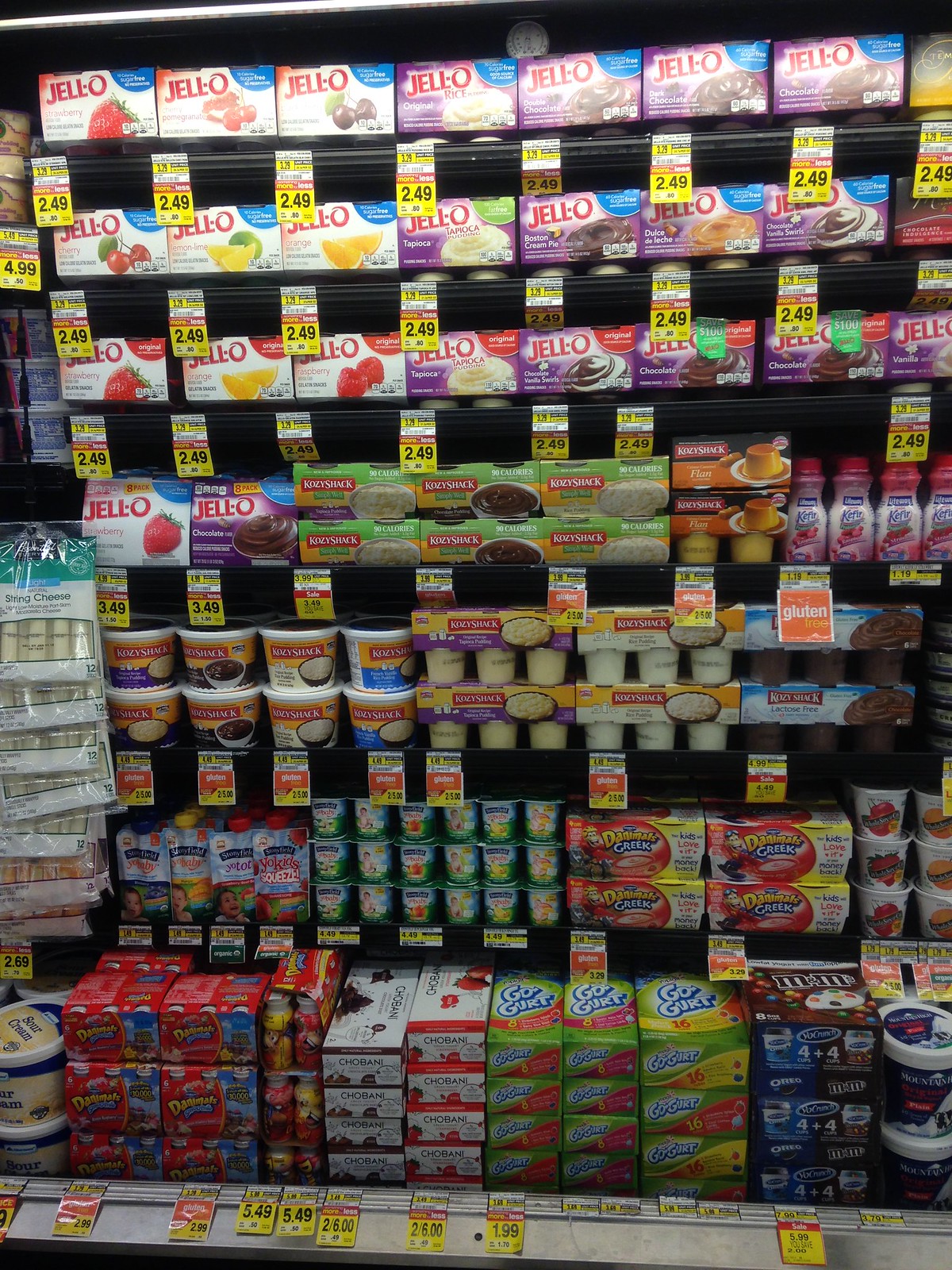This image depicts a detailed, close-up view of a refrigerated aisle in a grocery store, specifically an aisle featuring an extensive variety of chilled snacks. The section boasts six to seven shelves brimming with various brands of Jell-O products in multiple flavors and types, such as strawberry gelatin and chocolate pudding. Alongside the Jell-O, you can also find a range of Go-Gurt tubes in colorful, multicolor boxes, standing out prominently with green, red, and white packaging. There are tubs of rice pudding, alongside other snack offerings like drinkable yogurt and flan. Each level is meticulously organized, with yellow price tags affixed prominently to the shelves. The lowest level on the right corner features a unique M&M-themed refrigerated snack in a brown container. Additionally, the aisle includes specialized labels, such as an orange sign indicating gluten-free options.